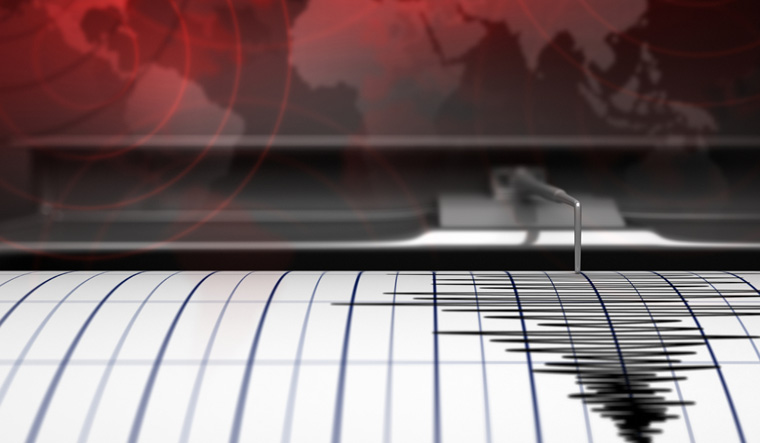This close-up image depicts a polygraph test in action. The primary focus is a slightly curved white sheet of paper, viewed from an angle just above it, which reveals an actively drawn graph featuring a grid of blue lines. A metal stylus, positioned on the left part of the photograph, extends and bends down to the paper, creating black lines that traverse from left to right across the graph. The background, occupying the upper portion of the image, is somewhat indistinct, reminiscent of a news studio setting with different shades of red and gray. Notably, there is no text present in the entire image, and the scene could be set in an office, a research facility, or might simply be a stock photo illustrating polygraph activity.